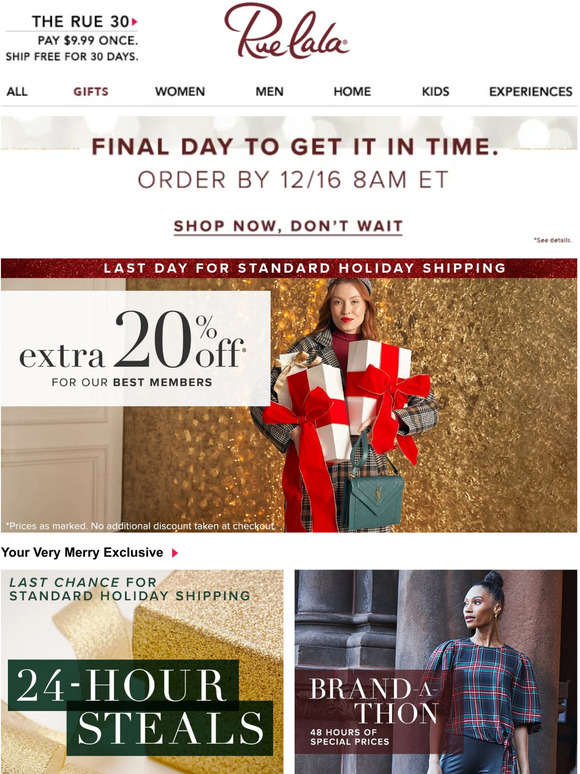A vibrant, screenshot-based promotional ad for Rue La La is shown, bursting with holiday shopping details. At the top left, there's text displaying "RUE" in three variations: "RUE" and "R-U-E." Adjacent to this is the bold “30” underlined with “RUE 30,” followed by a red arrow pointing towards the right. Below, a banner highlights a limited-time offer: "Pay $9.99 once and then ship free for 30 days."

Prominently placed in the center top is the Rue La La logo. Just beneath, a navigation bar categorizes shopping options into "All gifts, Women, Men, Home, Kids, Experiences," with "Gifts" currently highlighted. 

Midway down the page, a predominantly white and light gray segment informs shoppers: “Final date to get it in time,” emphasized by a directive: “Order by 12.16, 8 a.m. Eastern Time.” A call to action, “Shop now, don’t wait,” is underlined for urgency.

The central visual features a woman clad in a cozy, thick sweater, joyfully holding two white gift boxes adorned with red bows, underlined by the message “Last day for standard holiday shipping.” Further to the left, an alluring deal for the top customers reads: “Extra 20% off for our best members,” followed by a disclaimer in a small white font explaining, “prices as marked. No additional discount taken at checkout.”

At the bottom, two square screenshots capture ongoing sales events: "Last chance for standard holiday shipping, 24-hour steals" on the left, and "Brand-a-thon, 48 hours of special prices" on the right, ensuring that shoppers are acutely aware of the fleeting, valuable deals available. The entire setup encapsulates the urgency and excitement of festive shopping at Rue La La.